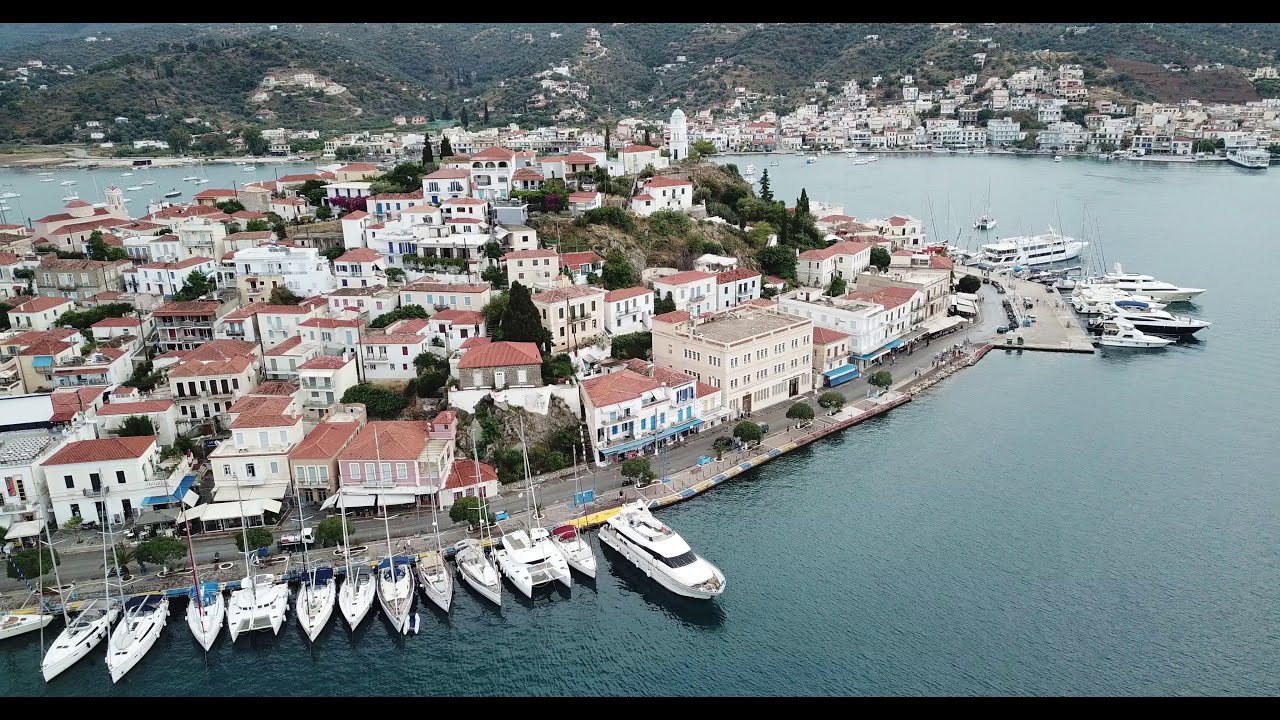This image depicts a picturesque European port city, likely resembling Mediterranean locales such as Greece or Italy. The scene is dominated by a hill-covered island surrounded by calm, light blue water. This main island, populated with numerous houses, features white facades and maroon-colored tiled roofs, creating a uniform aesthetic. At the pinnacle of the hill stands a unique structure, possibly a church, distinguishable by its spire and differing roof color. Luxury boats, sailboats, and personal yachts are moored around the island, adding a touch of opulence. A road can be seen leading down towards the water, enhancing the quaint charm of the area. In the distance, another lush, verdant hillside slopes upwards from the shoreline, adorned with more houses, reinforcing the impression of an idyllic waterfront community. The entire scene is bathed in daylight, amplifying the vibrant hues of blue, white, yellow, red, orange, tan, and gray present in the surroundings.